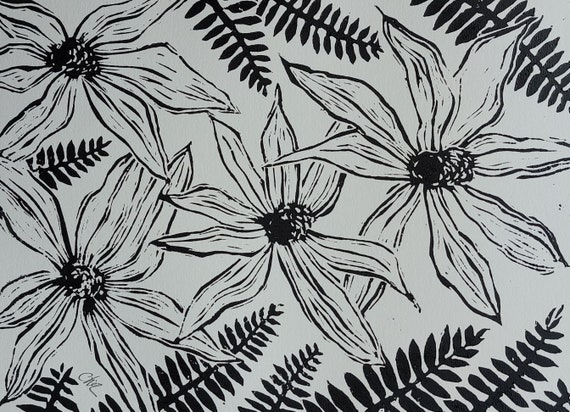The image is a monochromatic, black-and-white sketch on a dark grey or white background, featuring an intricate arrangement of jungle foliage and flora. Dominating the center are four star-shaped flowers, each with eight slender, elongated white petals radiating outward from a black, spotted ovary. These central flowers are framed by dark, fern-like leaves and branches, which extend uniformly from a main stem. The leaves form a ribcage-like pattern above and below the flowers, emphasizing the symmetrical and balanced composition of the scene. The artwork is two-dimensional, with no added depth or shading, giving it a simple yet striking appearance. The edges of the image are cropped, enclosing the detailed interplay between the flowers and the fern leaves within the limited space.